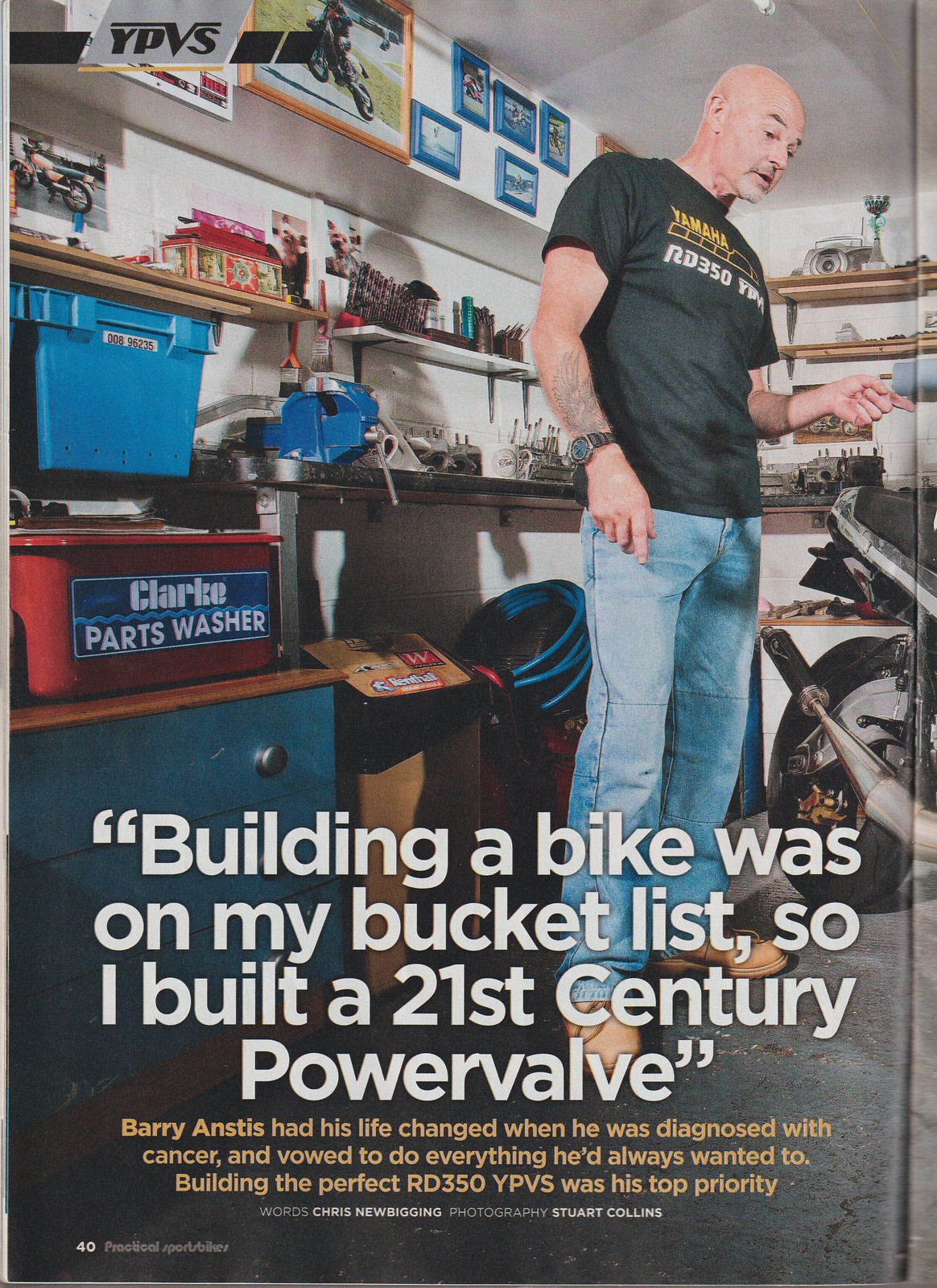In a magazine spread, the image features a middle-aged man standing in his garage, which has a concrete floor. The man is centered in the image and is dressed in a black t-shirt with yellow and white print, blue jeans, and light brown shoes. Surrounding him are shelves filled with various tools, toolboxes, and other storage items. The lower left center displays a red container labeled "Clark's parts washer," with a blue container above it and small house models further up. On the right side of the image, the man points to the back wheels and exhaust pipes of a motorcycle with his left hand. The caption at the bottom of the image reads, "Building a bike was on my bucket list so I built a 21st century power valve." In smaller gold print below, it states, "Barry Anstis had his life changed when he was diagnosed with cancer and vowed to do everything he'd always wanted to do. Building the perfect RD350 YPVS was his top priority." The background includes a detailed array of colors such as black, white, tan, gray, blue, light blue, red, yellow, orange, pink, and purple.